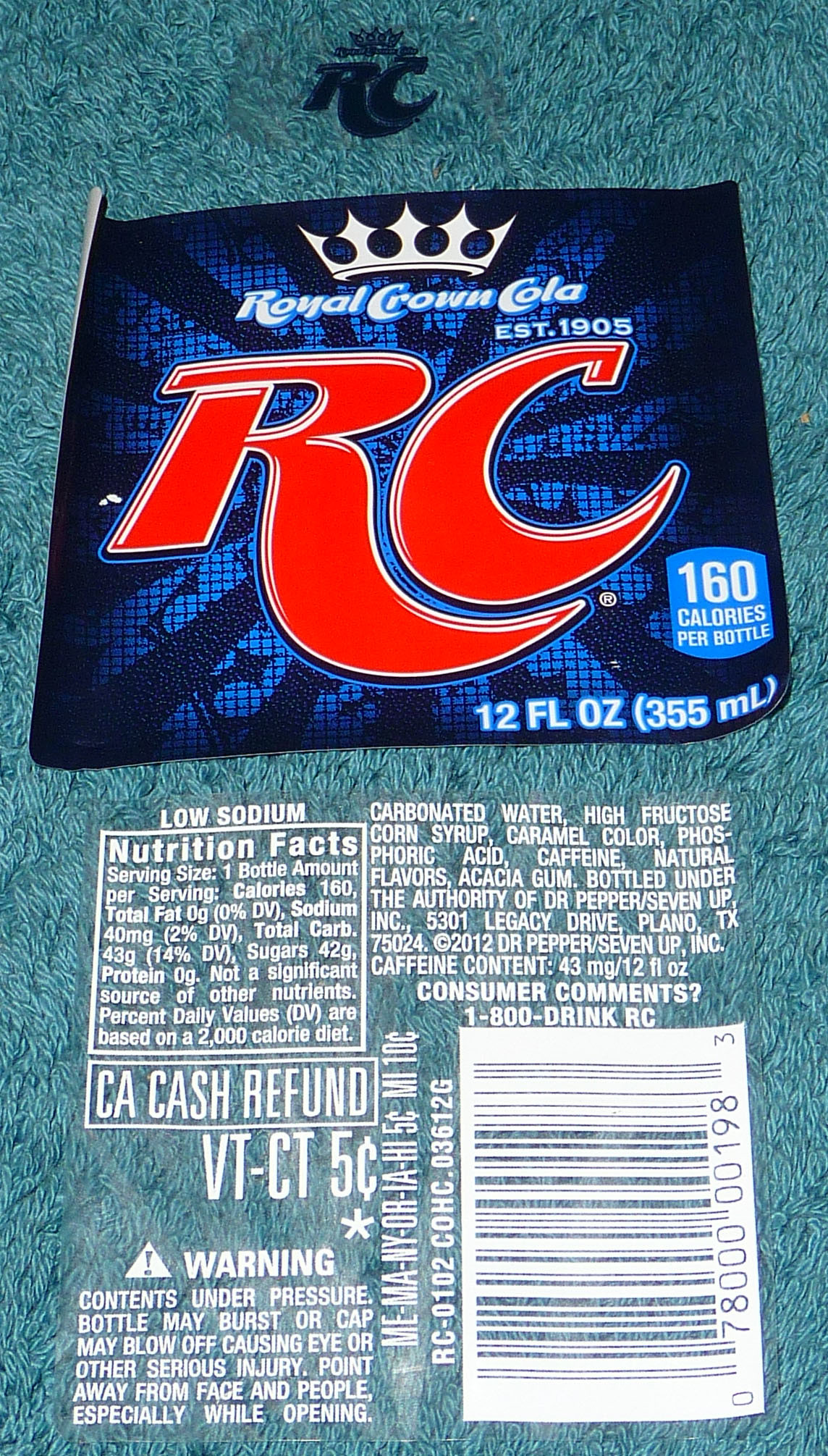This image captures a detailed view of an RC Cola label against a textured teal background, reminiscent of a short carpet or shag rug. The central feature is the RC Cola branding, prominently showcasing "RC" in bold red letters. Above this, in smaller white text, are the words "Royal Crown Cola" along with a depiction of a white crown, signifying the brand's heritage. The label also notes "Established 1905" and specifies the drink's volume as "12 fluid ounces (355 milliliters)". This information is situated on a starburst design, radiating from a medium blue center to a darker blue outer edge, creating a striking visual against the teal backdrop.

Below the main branding, the image provides detailed product information including nutritional facts (such as 160 calories per bottle), ingredients (carbonated water, high fructose corn syrup, caramel color, phosphoric acid, caffeine, natural flavors, and acacia gum), and a cautionary label about the potential for the contents to burst. Additionally, it lists the address of the bottling authority, Dr. Pepper 7-Up, at 5301 Legacy Drive, Plano, Texas.

This photograph appears to capture multiple labels from an RC Cola can or bottle, laid out on the textured teal surface, giving an effect reminiscent of memorabilia or promotional items.